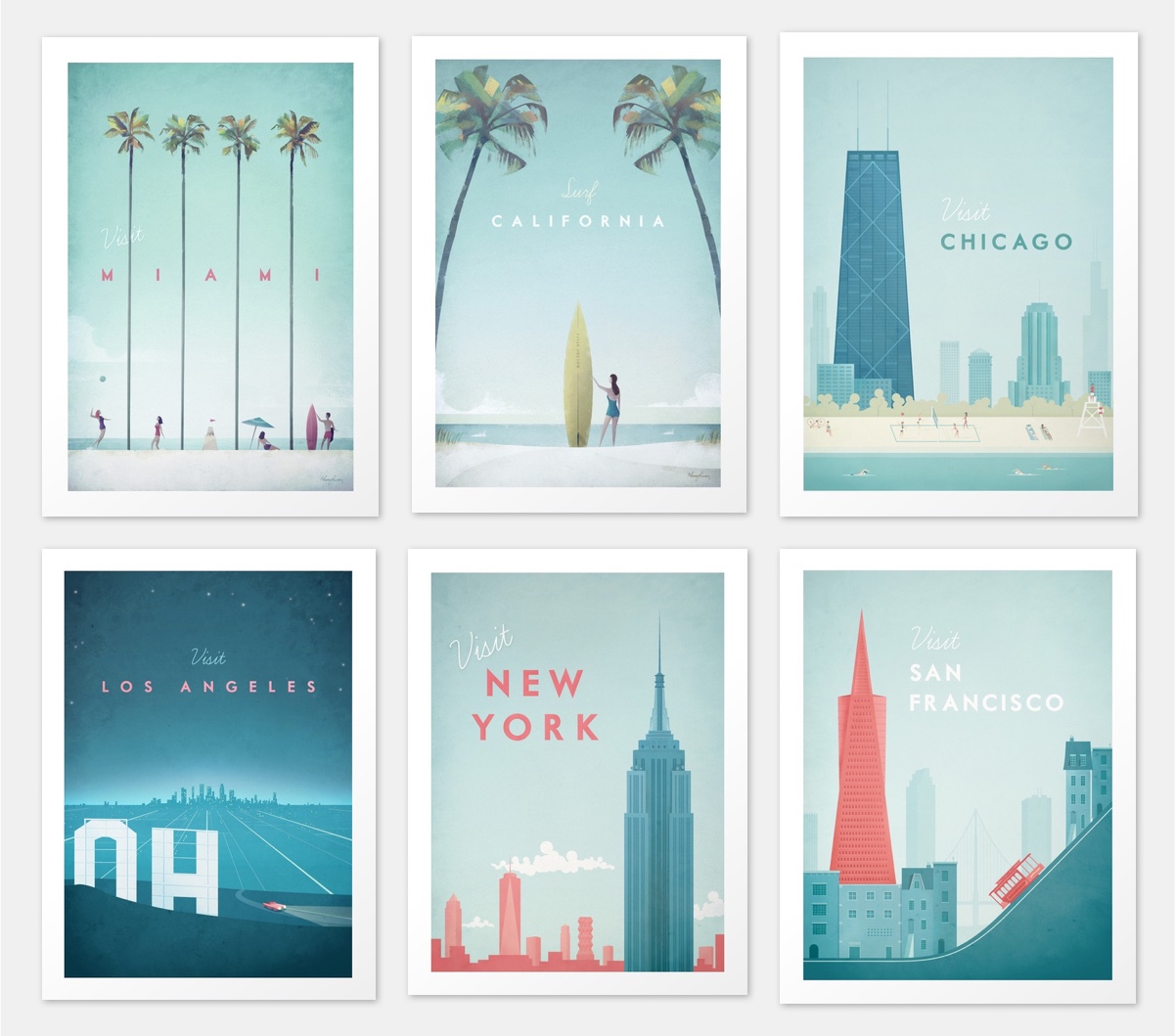The image showcases six posters arranged in two rows, each representing a different city with a shared, cohesive cartoon style reminiscent of graphic designs found in Ikea. Each poster is bordered in white and employs a palette predominantly featuring light and dark blue, with accents of green, reddish-pink, and light yellow.

In the top left poster, "Miami" is spelled out between four tall palm trees on a white sandy beach with a strip of sea in the backdrop. The scene includes four people engaged in beach activities, including one holding a surfboard and another with an umbrella. Moving to the middle top, the "California" poster features a woman standing with a surfboard flanked by two palm trees. 

The top right poster advertises "Visit Chicago" with a skyline viewed from the sea, showcasing tall buildings and a sandy foreground. On the bottom left is a night-time scene titled "Visit Los Angeles." This poster captures a fragment of the iconic Hollywood sign against a dark sky. 

In the center bottom is "Visit New York," prominently displaying the Empire State Building amid other skyscrapers. Lastly, at the bottom right, the "Visit San Francisco" poster depicts a classic hill with a trolley climbing up, with various buildings in the background. Each poster vividly captures the essence of its respective city through unique, yet harmoniously styled illustrations.